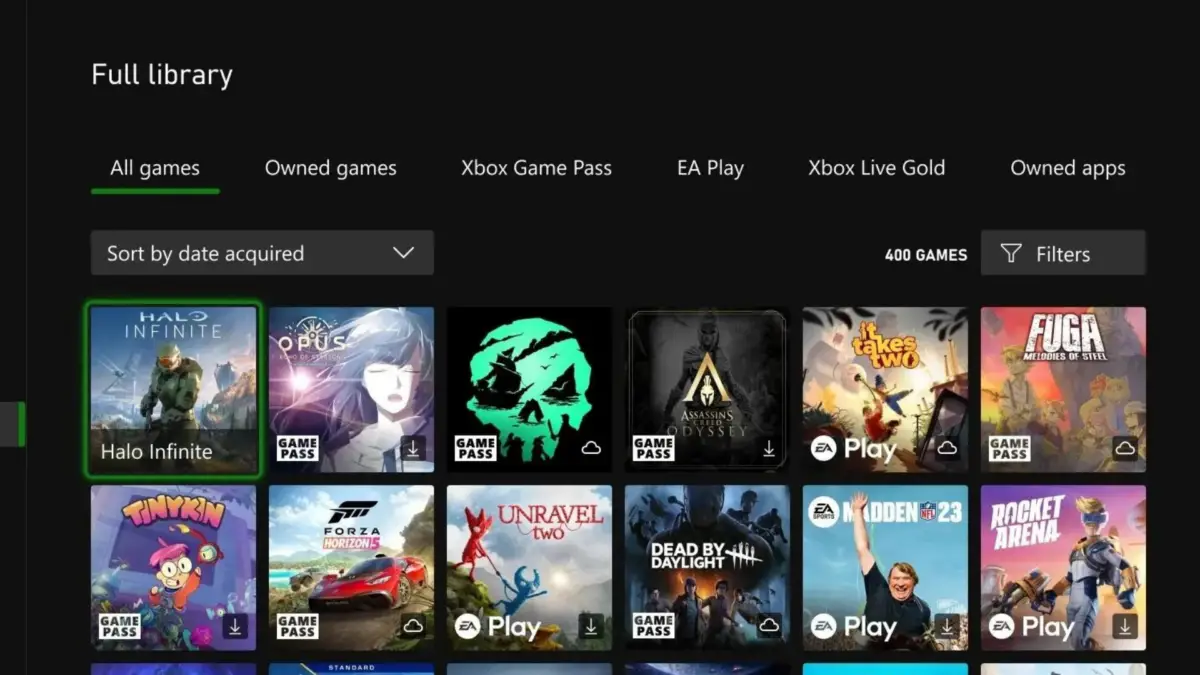This image captures the detailed interface of a gaming library web page set against a black background. In the top left corner, the heading "Full Library" is displayed prominently in white text, indicating that this is a user's comprehensive collection of games. Directly below the heading is a horizontal navigation bar with various sorting options, such as "All Games" (which is currently selected), "Owned Games," "Xbox Game Pass," "EA Play," "Xbox Live Gold," and "Owned Apps."

Further down, a drop-down menu labeled "Sort by Date Acquired" allows users to organize their game collection. Adjacent to this menu, a filter option provides users with the ability to further refine their selection, noting that there are a total of 400 games in the library.

The main content is displayed in two horizontal rows of game thumbnails, each with its corresponding cover image. The first row includes titles such as "Halo Infinite," "Opus," and another game featuring a neon green skull on a black background, all marked with the "Game Pass" label. Following these are "Assassin's Creed Odyssey" (also marked with "Game Pass"), "It Takes Two" (labeled "EA Play"), "Fuga: Melodies of Steel" (also marked "Game Pass"), and "Tinykin."

Below the first row, the second row features games like "Forza Horizon," "Unravel 2," "Dead by Daylight," "Madden NFL 23," and "Rocket Arena." There are additional games visible further down the list, but they are cut off at the bottom edge of the image, indicating that the library contains even more content ready for exploration.